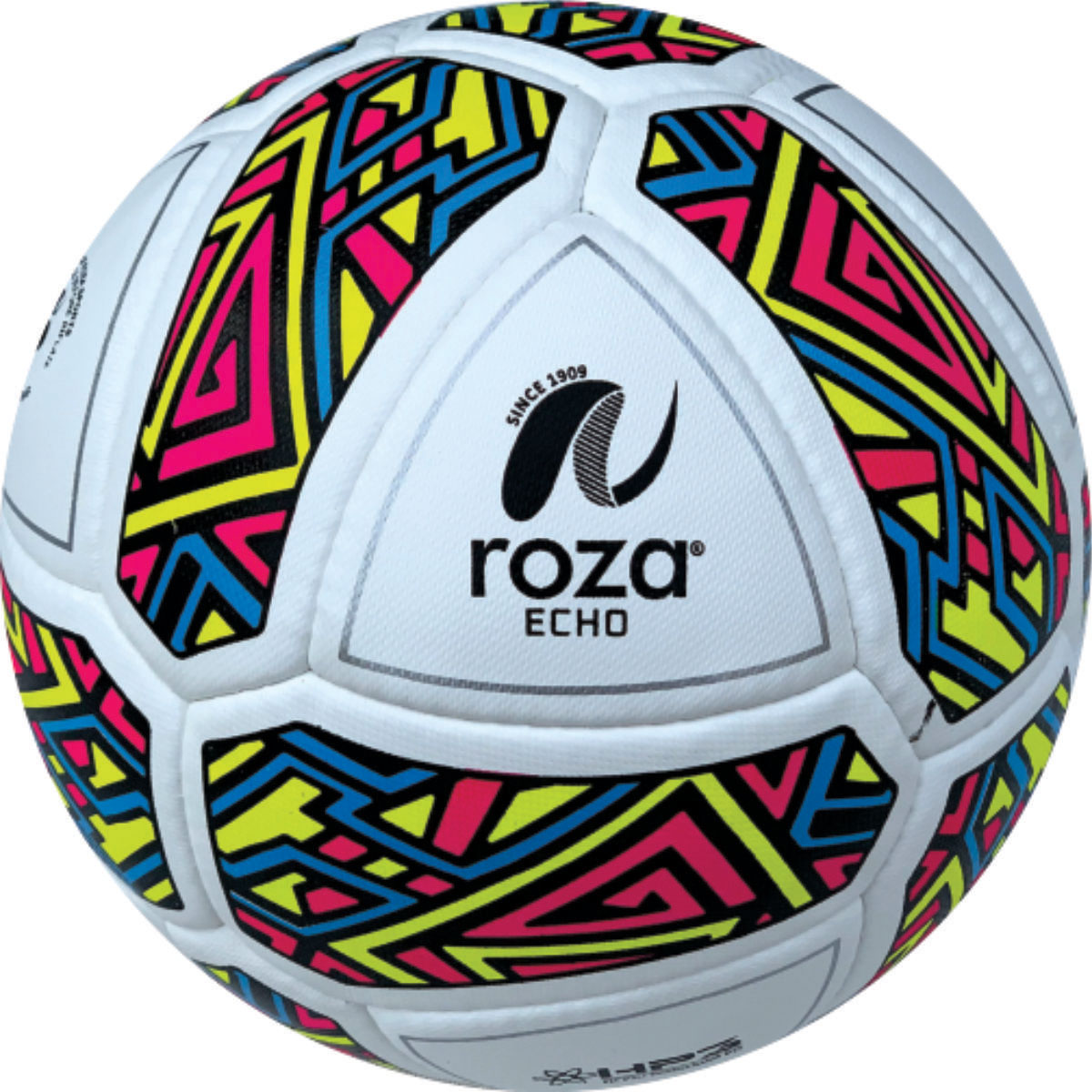This close-up image showcases a soccer ball with a detailed and colorful design. The ball features multicolored geometric patterns consisting of squares, triangles, and lines in blue, yellow, red, and black, all separated by white seams and stitching. Prominently displayed on one of the panels is a black curved triangle with a logo or insignia inside, followed by the word "ROZA," spelled R-O-Z-A, and "ECHO" in smaller capital letters beneath it. The logo is emphasized with the text "Since 1909." Surrounding this, various panels contain intricate geometric designs, with certain white panels featuring additional black writing or insignias. The overall design lacks a set pattern but is carefully sectioned by black outlines. The background of the image is entirely white, highlighting the ball and making the detailed multicolored designs stand out even more.